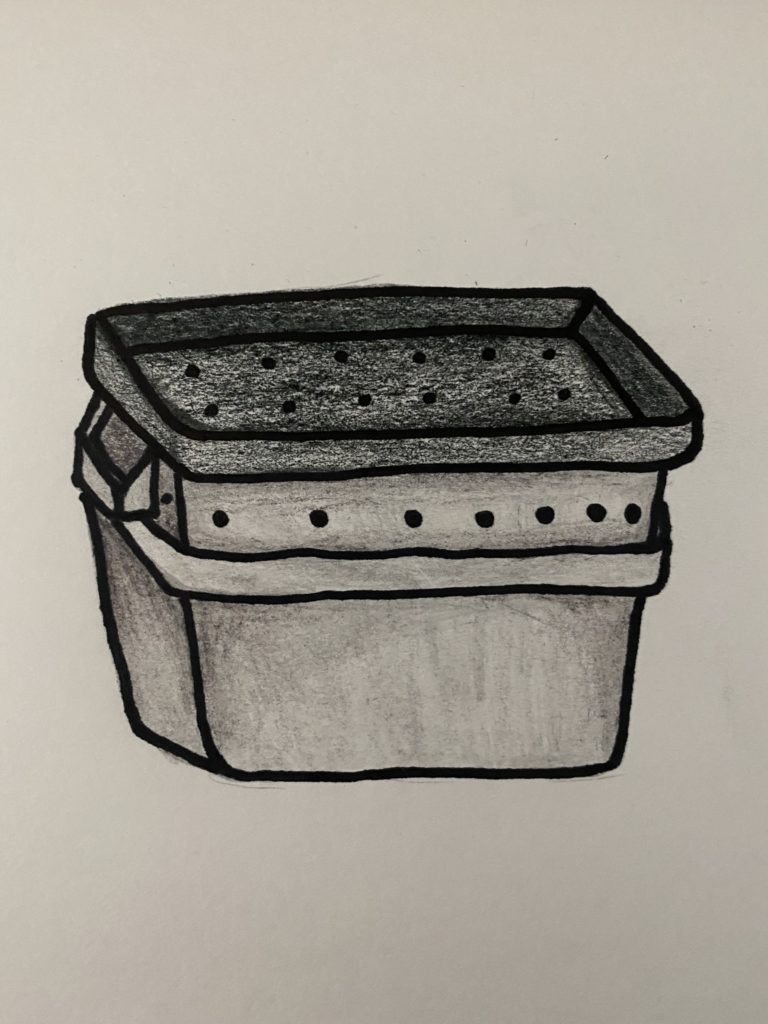This image is a detailed drawing created using what appears to be a black marker or thin black pen, possibly complemented by charcoal or crayon for shading in shades of black and gray. The illustration depicts a box-shaped object with a classic rectangular bottom. Above the bottom section, there is a broader compartment resembling a cooler or a ventilated container, potentially from an older era. The top portion of this object features a lid dotted with around 12 to 14 small black spots, likely representing holes meant for ventilation. Additionally, there are seven black spots arranged on the upper section, spaced a few inches apart, hinting at further air vents. The presence of a handle on the left side of the structure suggests it is something that can be carried, possibly designed to transport living things or items that require ventilation. The overall appearance and construction of the object leave its exact purpose open to interpretation, but it could be perceived as either an antiquated cooking device, a ventilated container, or even an old-fashioned garbage receptacle.